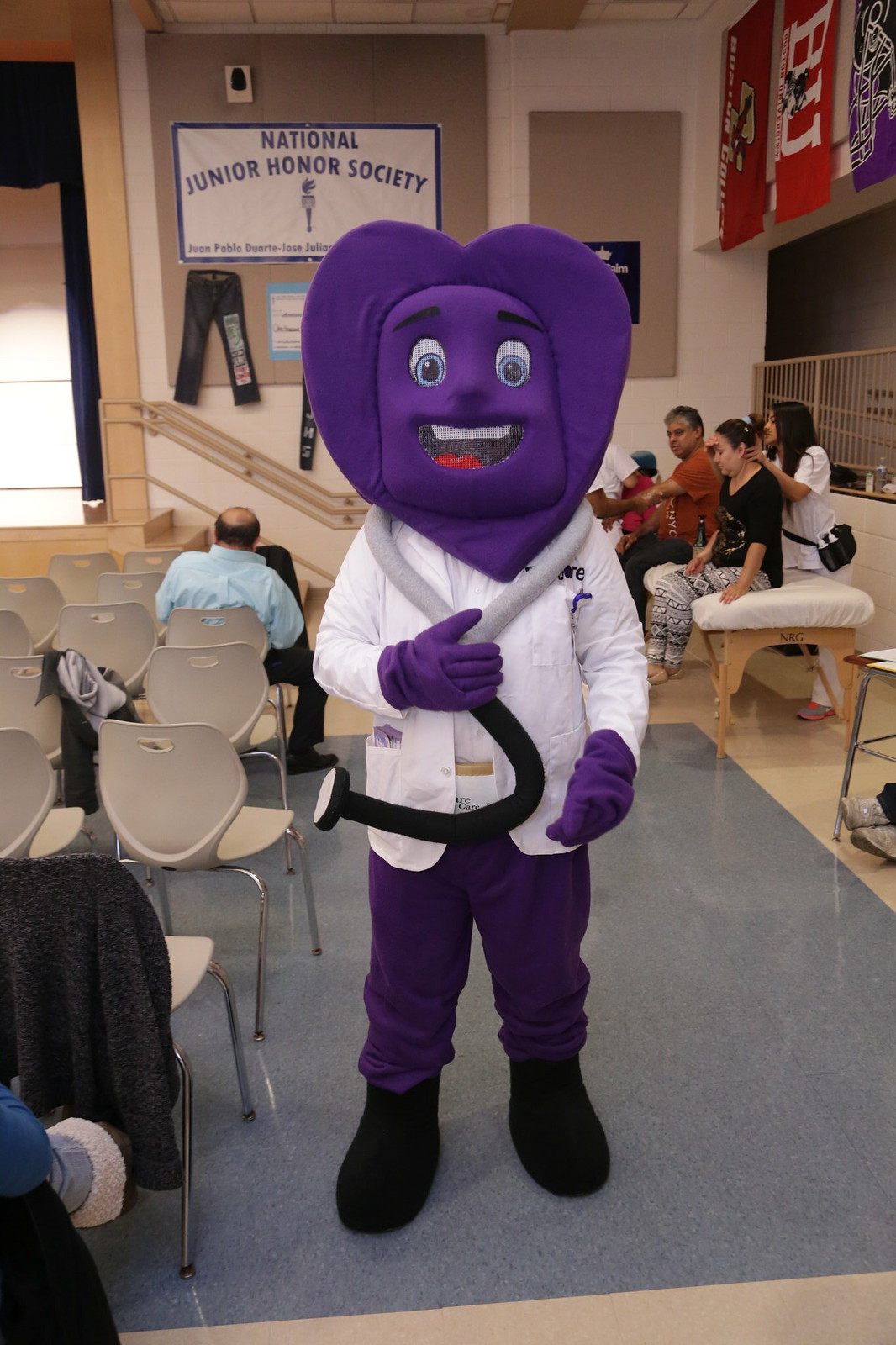In this image, a costumed character stands front and center in what appears to be an auditorium or a cafeteria outfitted with chairs and a small stage. The back wall displays a "National Junior Honor Society" flag, indicating a scholastic setting. The mascot itself has a striking appearance with a heart-shaped, purple face framed by a mane-like structure and large blue eyes. Its mouth is open, revealing teeth and a tongue. Dressed in a white doctor's coat and purple pants, the character also sports purple gloves, black shoes, and a large, exaggerated stethoscope around its neck. To the right, a scene unfolds where individuals look to be engaged in health-related activities; one woman is being examined, possibly for a headache, while another man seems to be preparing to give blood. The light brown and blue tiled floor adds to the quaint, community-focused atmosphere of the setting.